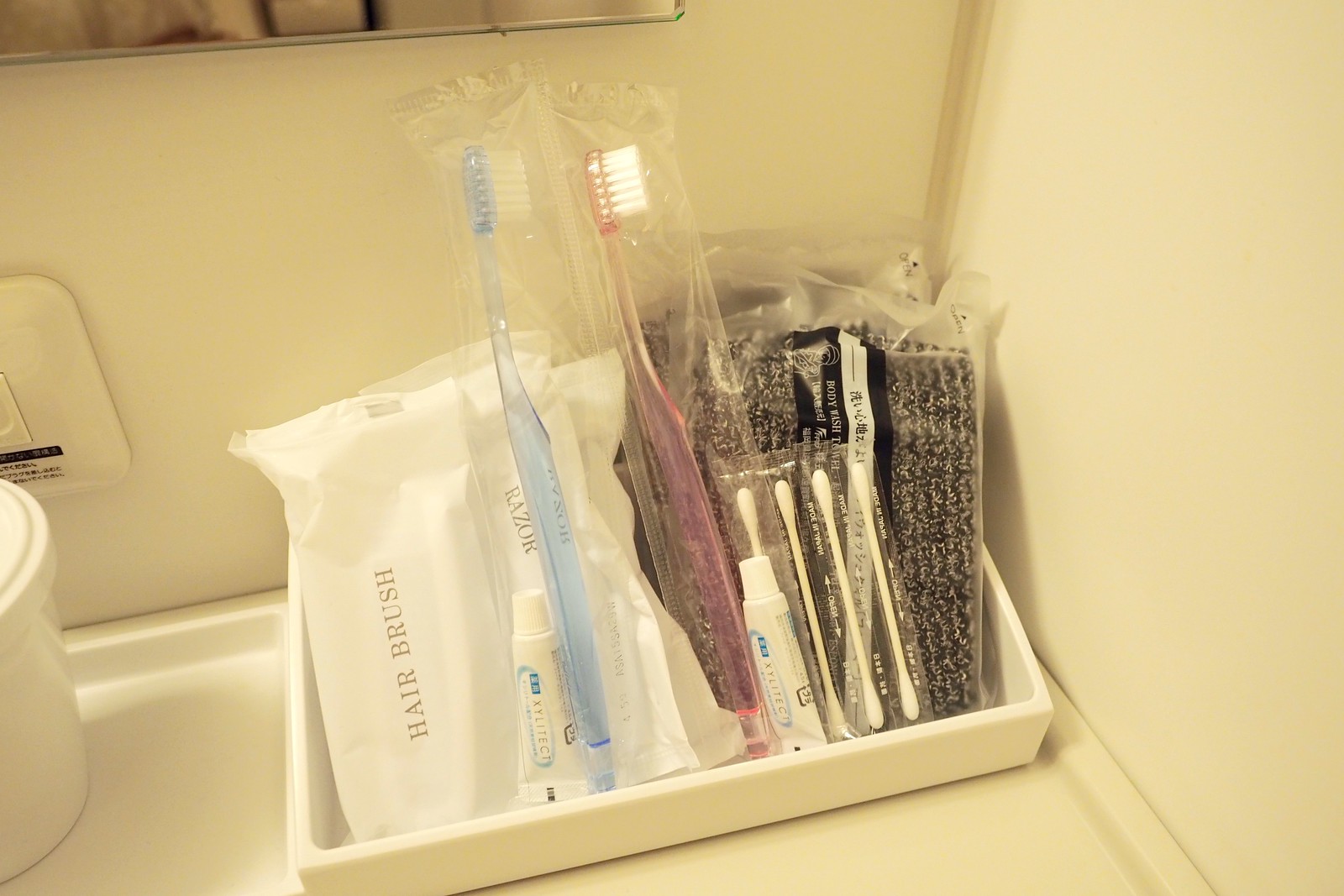This detailed, landscape-oriented photograph depicts a high-class hotel bathroom amenity tray, embodying elements of Japanese hospitality. Positioned on a bathroom counter, this white tray holds an array of neatly packaged toiletries, each clearly labeled in Japanese kanji. The offerings include a blue toothbrush and a pink toothbrush, both accompanied by small white tubes of toothpaste. Also visible is a plastic-wrapped hairbrush, a razor, and miniature containers of Q-tips (four in total). Additionally, the tray contains hair ties, a body wash, and what appears to be a rough cloth for exfoliation. The scene is illuminated by warm, yellow lighting, enhancing the inviting appearance of these meticulously arranged amenities.